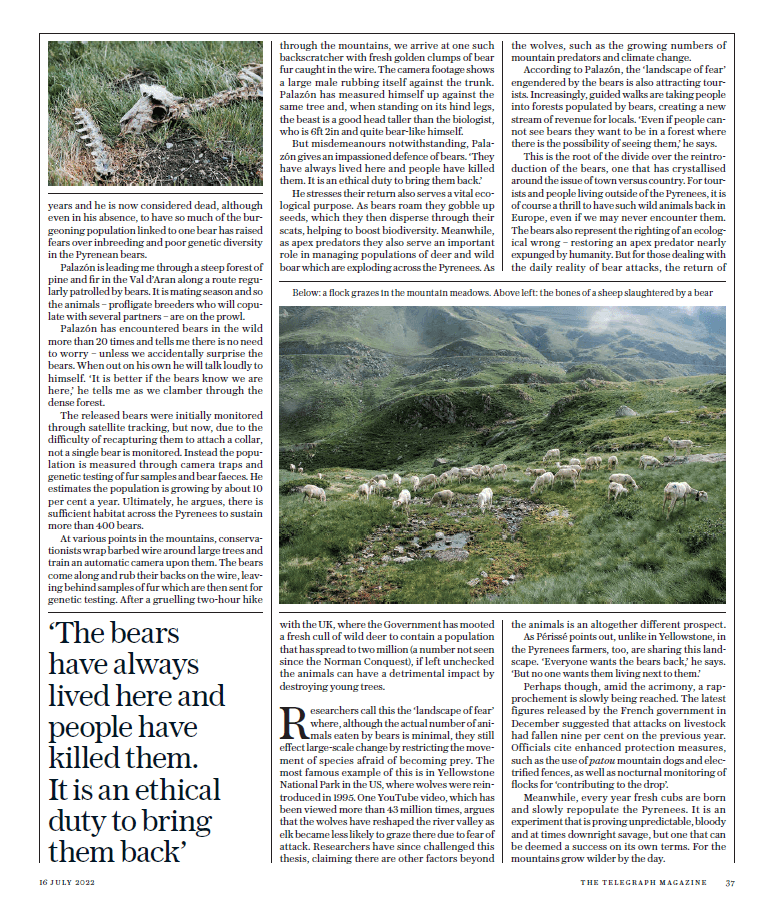This image portrays a news article displayed on a computer monitor, sourced from The Telegraph magazine, dated July 16, 2022, specifically from page 37. The photograph includes two distinct images. The first image, located above the left section, depicts the skeletal remains of a sheep, laying on unkempt grass indicative of a recent encounter with a predator, likely a bear. The second image, centrally positioned, features a flock of sheep peacefully grazing in lush, fertile mountain meadows. The surroundings suggest a remote, mountainous area abundant in greenery, far removed from urban locales.

Accompanying these images is text that provides context: "Below, a flock grazes in the mountain meadows. Above left, the bones of a sheep slaughtered by a bear." Further, a poignant quote emphasizes the article's theme: "The bears have always lived here, and people have killed them. It is an ethical duty to bring them back." This caption not only identifies the locations and subjects of the photographs but also hints at a broader, possibly conservation-focused narrative concerning the coexistence of local wildlife and human activities.